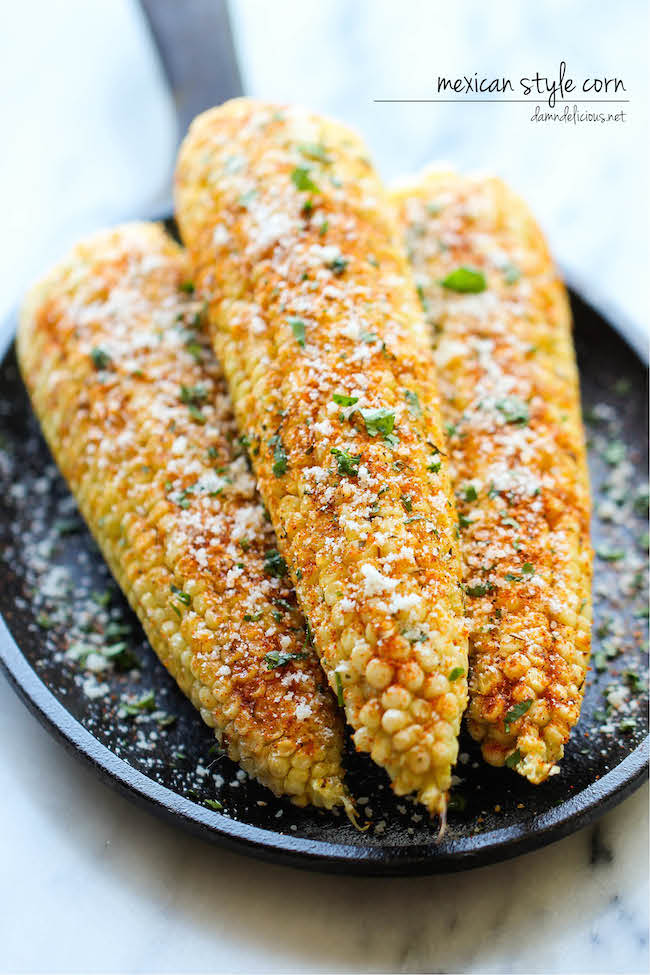This image showcases a dish of Mexican-style corn, known as elote, arranged on what appears to be a large, black cast iron skillet with a long handle facing away and upwards from the camera. Positioned vertically with two ears of corn on the bottom and one on top, the roasted corn cobs are dusted with a combination of seasonings. Garnished with what seems to be crumbled parmesan or cotija cheese, black specks possibly of cilantro or onion, and hints of red seasoning akin to pepper or a Cajun spice blend, the corn is slightly browned at the ends, indicating a well-roasted preparation. The skillet rests on a marbled surface of gray, white, and black hues, adding to the aesthetic appeal of the presentation. The upper left corner bears the text "Mexican-style corn" in black, with a caption below suggesting "simply delicious." The image also points to being sourced from "damndelicious.net," conveying both the cultural authenticity and the tempting appeal of this traditional Latin American dish.